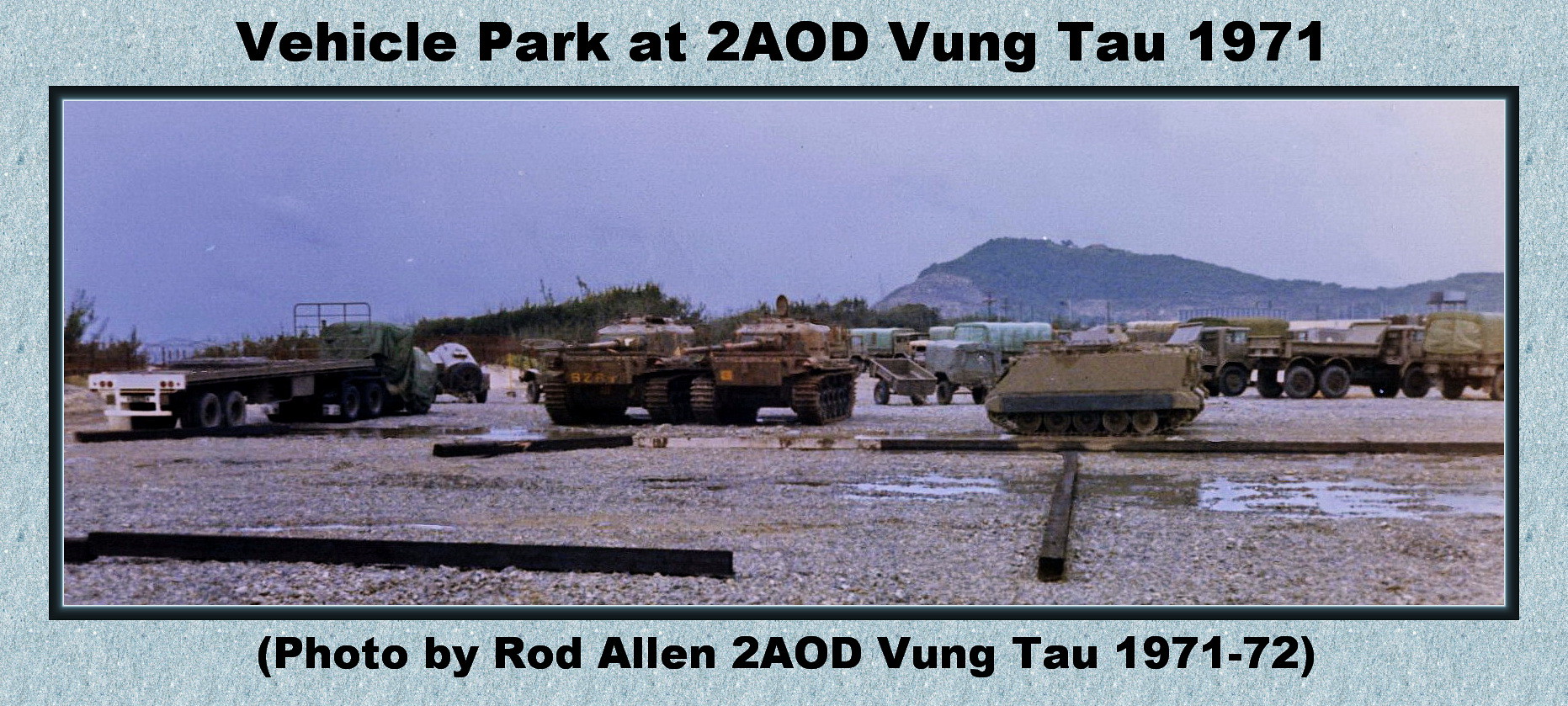The image depicts an outdoor area during the Vietnam War era, specifically a vehicle park at 2 AOD, Vung Tau, in 1971. It features a variety of military vehicles, including several tanks, a few military trucks, armored personnel carriers, and a flatbed truck positioned on the left end. The landscape is mostly flat and gravelly, interspersed with wooden planks arranged in different directions. In the background, a distant mountain range and patches of greenery are visible under an overcast, hazy sky. The picture is framed within a black rectangular box with overlapping black font. The title at the top reads, "Vehicle Parked 2 AOD, Vung Tau, 1971," while the caption below credits the photo to Rod Allen and dates it from 1971 to 1972. The overall layout has a dark border between the picture and the mat, and the image was likely photographed on a concrete or rocky ground, contributing to its historical significance.